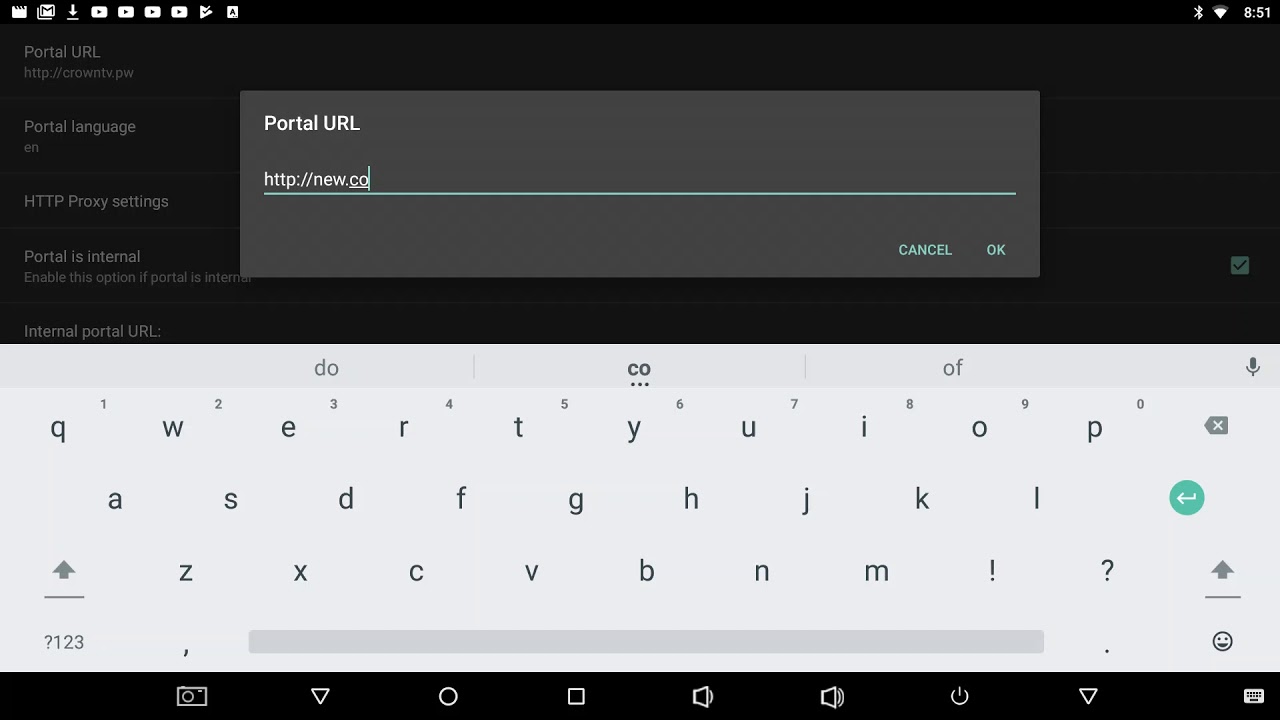The image displays a horizontal rectangular interface split into two distinct halves. The top half features a black background, within which lies a dark gray dialog box. In the upper left corner of this dialog box, “Portal URL” is written in white text. Below this, an incomplete URL, "http://new.co," is typed in white text, followed by a blinking cursor line, suggesting ongoing input. Positioned at the bottom right corner of the dialog box are two buttons, "Cancel" and "Okay," highlighted in turquoise.

Adjacent to the dark gray dialog box, on the left side of the black background, is a vertical list of menu options displayed in white text. The options include “Portal URL,” “Portal Language,” “HTTP Proxy Settings,” and “Portal is Eternal.”

The bottom half of the page transitions to a light gray background, which houses a virtual keyboard. The keyboard maintains a standard layout with letters positioned in their conventional places. At the very bottom of the screen, there is a thin black ribbon containing various icons, arranged from left to right.